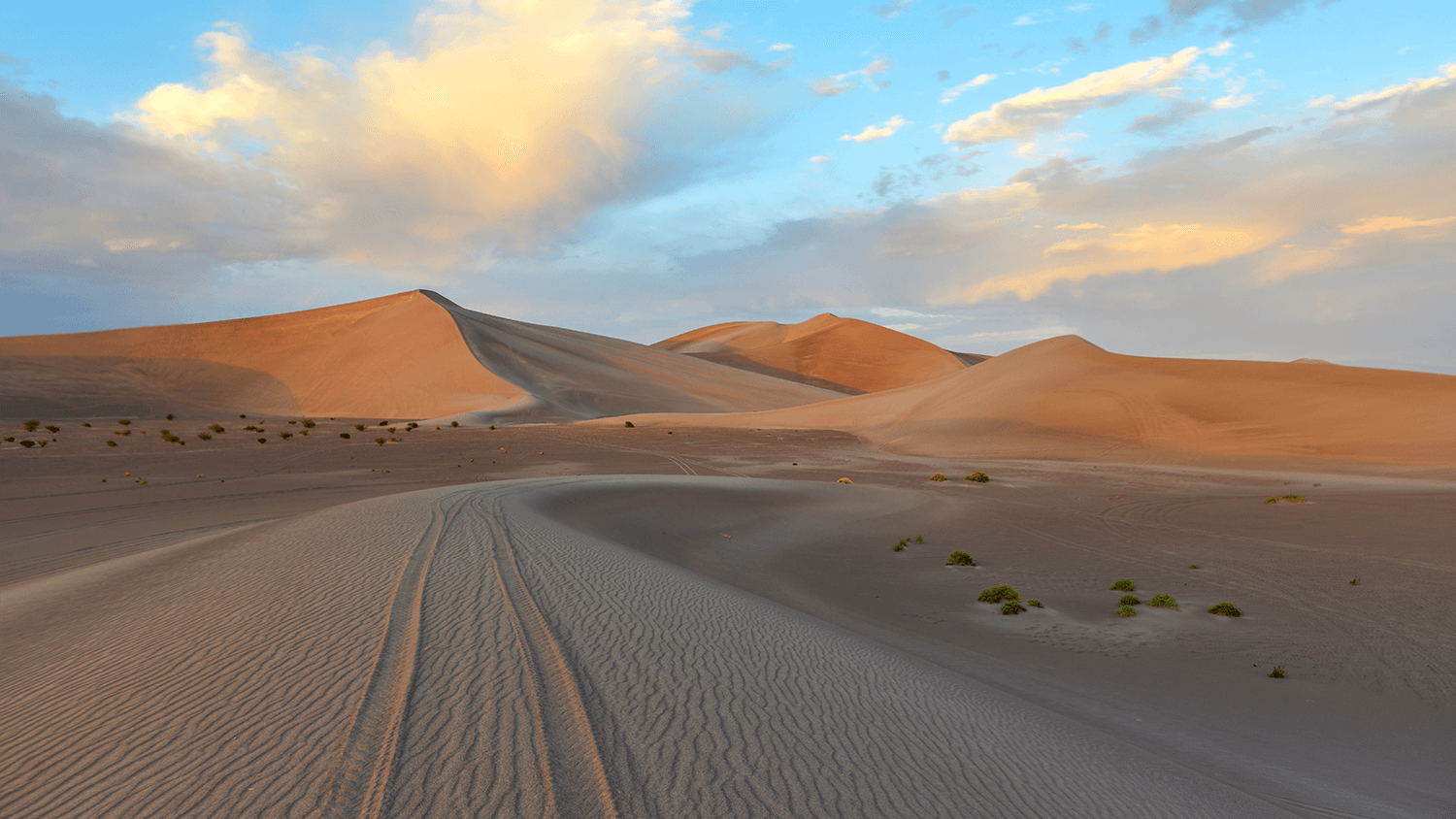The image captures a serene desert landscape during the day, showcasing an array of subtle yet stunning colors. The horizon sits halfway up the image, dividing a vivid blue sky filled with fluffy white clouds tinged with gray shadows from the sun's light. The sun appears to be casting a warm, golden glow that accentuates the rustic tan hues of the sand dunes.

Centered in the background are three prominent sand dunes. The largest dune dominates the left side of the picture, extending from the far left edge to the middle. Another dune peeks up from behind in the distance, adding depth to the scene. The third dune, closer and slightly smaller than the largest, overlays the others from the middle to the right side of the image.

In the foreground, a pair of parallel tire tracks winds from the lower left corner, curving right towards the horizon, suggesting a vehicle's recent passage. The tracks are embedded in a lower sand dune that leads the eye into the distance. The sand shows delicate wave patterns, hinting at windswept moments frozen in time. On either side of the tire tracks, sparse desert shrubs pepper the landscape. These bushes, some green and others with a reddish hue, provide a stark but beautiful contrast to the sandy terrain.

The overall scene exudes a still, crisp atmosphere with no visible haze or blowing sand, capturing the tranquil beauty of the desert.